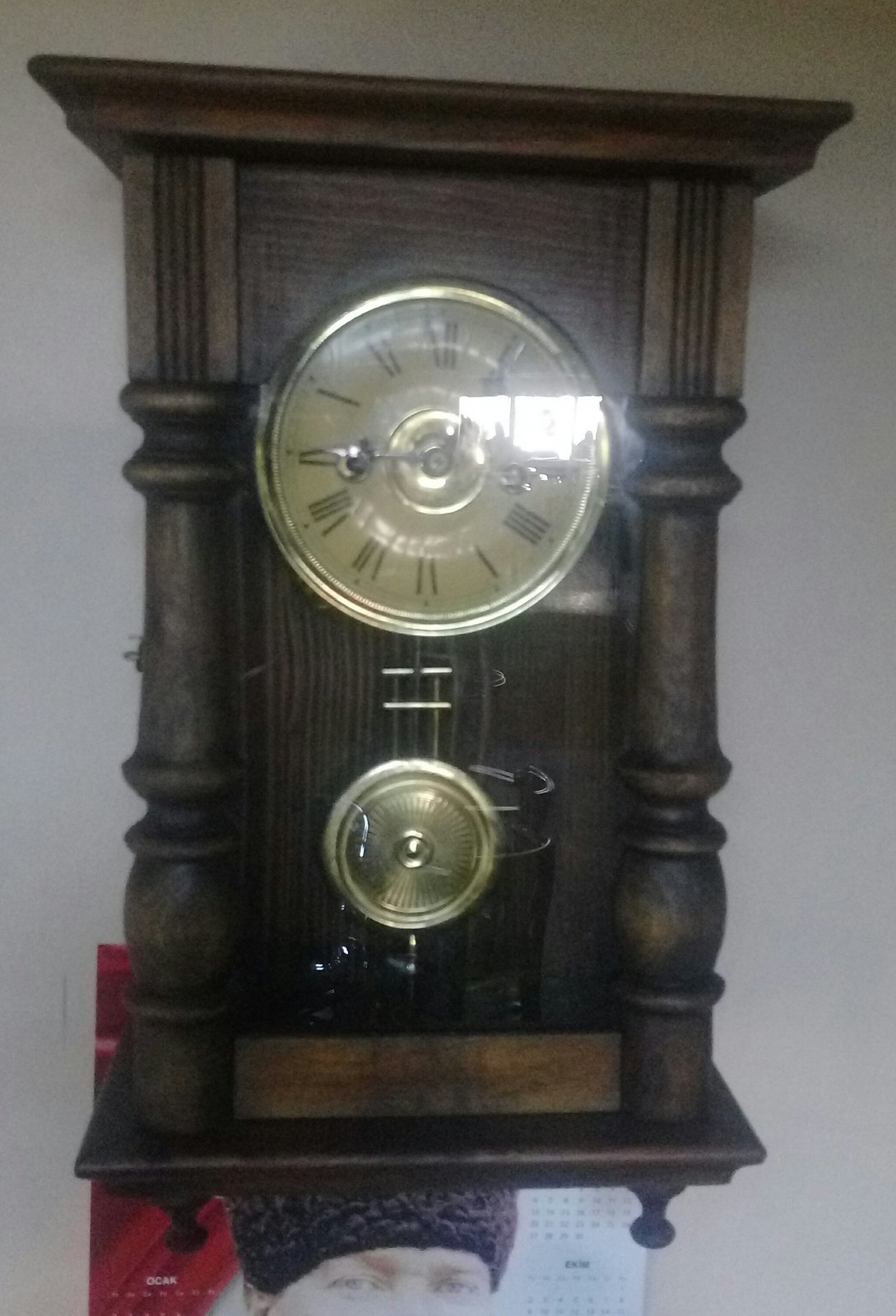This photograph captures a charming, antique-style clock with a wooden outer frame. The clock face features a vintage aesthetic, characterized by a yellowish-white background with Roman numeral markers. A golden-hued pendulum hangs elegantly below the main clock face. The timepiece is enclosed in a wooden case, and although a portion of a picture of a person is visible beneath the clock, it remains out of focus and largely off-screen, ensuring the clock remains the primary subject.